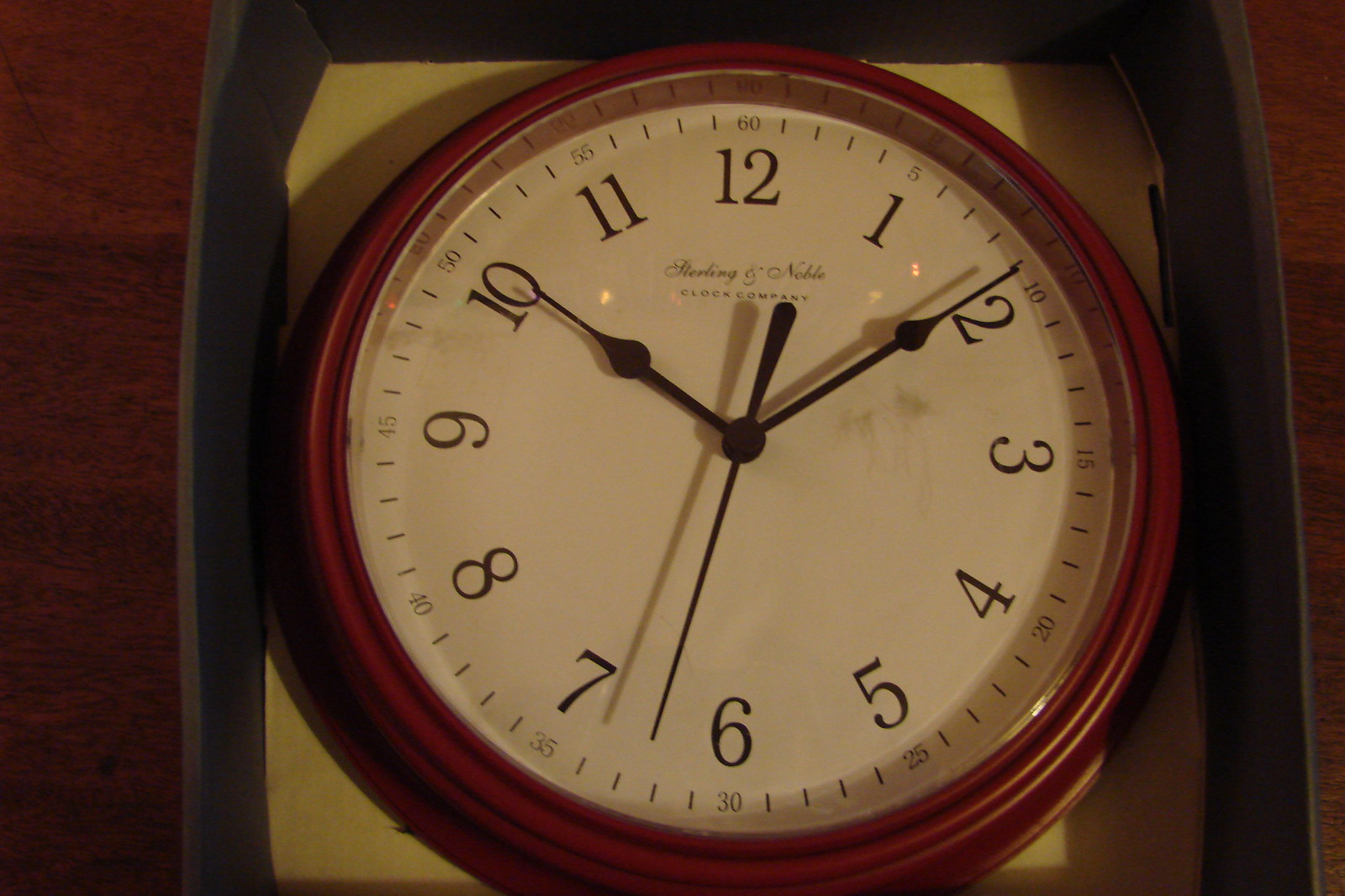The image showcases a clock encased in a dark-colored box with a white bottom. The clock features a reddish-brown wooden housing and a translucent plastic cover on the front. The clock face is white with black numerals and black tick marks signifying minutes. Each hour numeral is accompanied by a smaller numeral representing 5-minute intervals: 1 with 5, 2 with 10, 3 with 15, 4 with 20, 5 with 25, 6 with 30, 7 with 35, 8 with 40, 9 with 45, 10 with 50, 11 with 55, and 12 with 60. The face also bears the inscription "Sterling and Noble Clock Company." The clock hands—hour, minute, and second—are all black. The entire setup is placed on a dark brown wooden table.